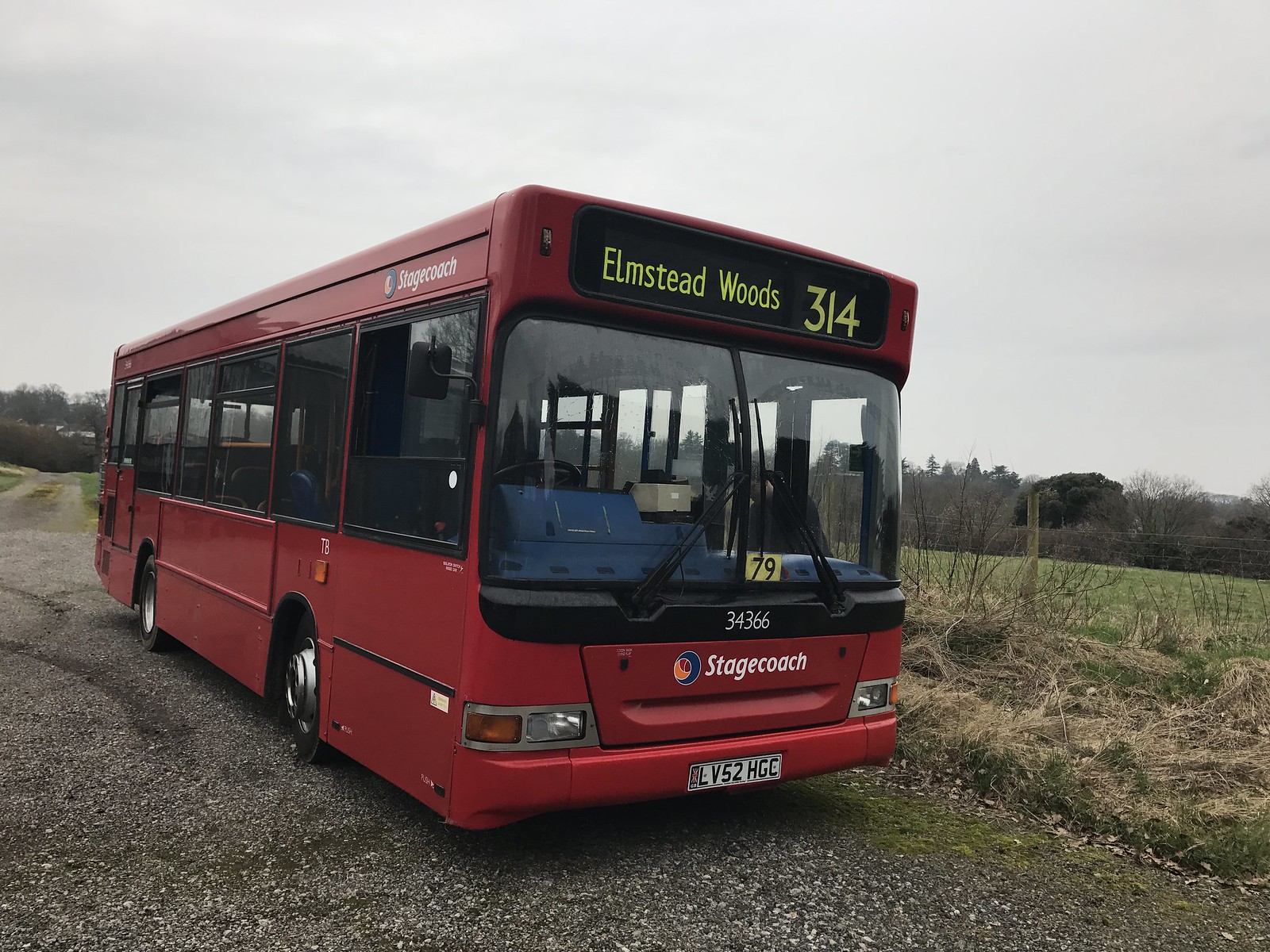The photograph depicts a large red Stagecoach bus parked on a gravel road in a rural setting. Positioned at a three-quarter angle facing to the right, the bus features a wide, flat windshield with black wipers and dark wide windows along its red shell. Above the windshield, a black sign displays "Elmstead Woods" in green letters and the route number "314". Below the windshield, "Stagecoach" is written in white italic letters across the grille, accompanied by a round orange and blue logo to the left. The license plate on the front bumper reads "Wiesenwichter 52 HGL" on a white background. Inside, blue seats are visible. The bus is surrounded by a field bounded by a wire fence, with a tree line in the distance under a gray, cloudy sky, making it appear as though it is parked in an isolated, countryside location.